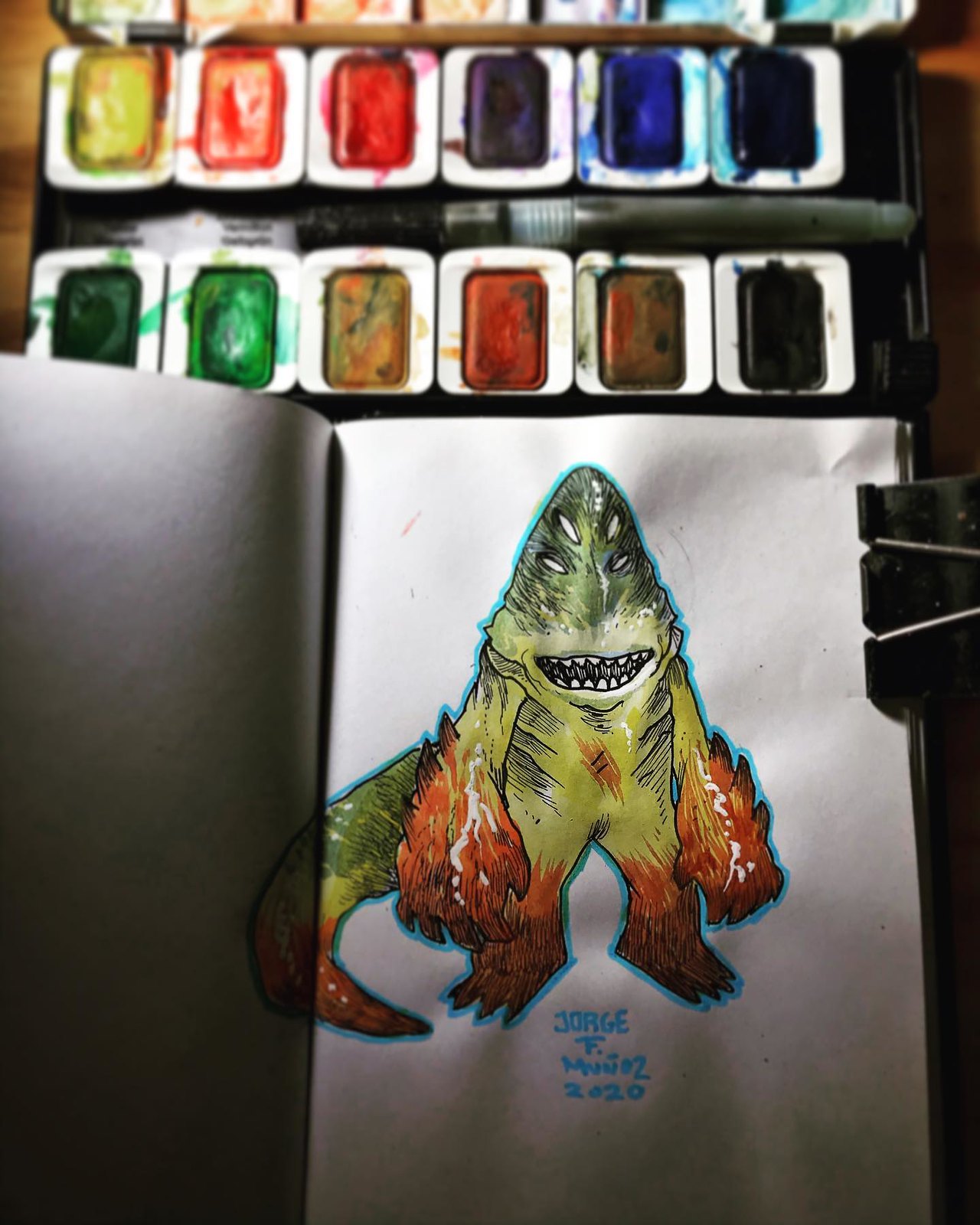The image depicts an open sketchbook lying on a surface with a black cover visible on the left side and a white page clipped with a metal binder clip on the right. On the white page, a detailed illustration of a green, chubby-bodied monster with a triangular, pointy head dominates the scene. The monster features four eyes arranged symmetrically on either side of its jagged, sharp-toothed mouth. Its arms taper into large hands that appear to be engulfed in fiery red and orange hues, similar to its feet and the tip of its tail. The forearms have prominent spikes adding to its menacing appearance. The illustration is outlined in blue, and below it, the artist's signature reads "Jorge F. Munoz, 2020."

Above the sketchbook, there is a well-used paint palette with multiple color wells. The palette's top row showcases an array of colors starting from yellow, orange, red, purple, blue, and dark blue or black. The bottom row contains a mix of dark green, lighter green, yellow, orange, mixed shades of yellows and oranges, reds, and another dark hue that looks like black. The palette is notably messy, indicating frequent use.